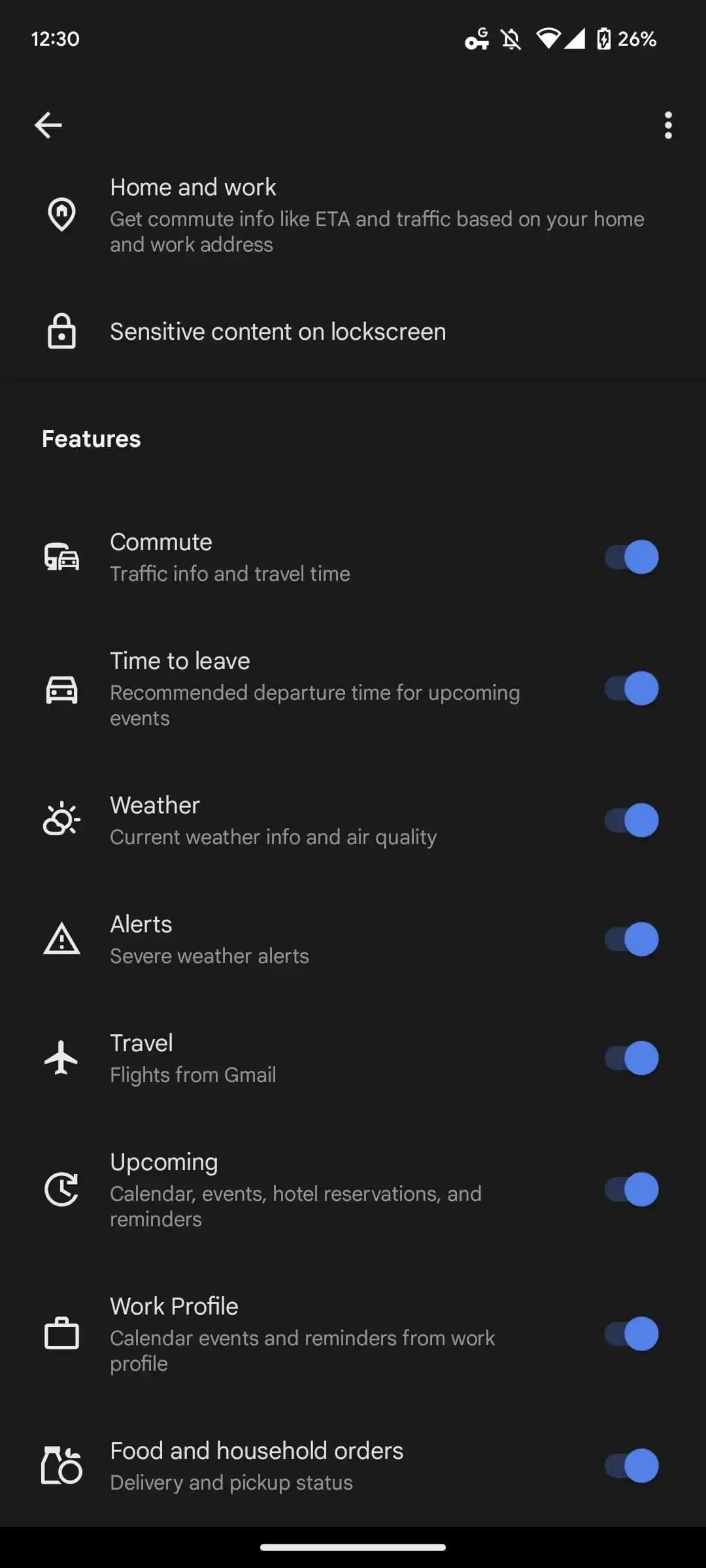This image showcases a comprehensive all-in-one assistant app integrated into the operating system, characterized by a sleek dark background and white text providing a clear, high-contrast interface. The screen prominently displays multiple settings categories, each focused on enhancing user convenience. Key sections include:

- **Home and Work**: Offers commute information, such as ETA and traffic conditions, tailored to the user's home and work addresses.
- **Sensitive Content on Lock Screen**: Manages what is shown when the device is locked.
- **Commute**: Provides updates on the best times to leave, live traffic updates, and alternate routes for daily commutes.
- **Features**:
  - **Time to Leave**: Recommends departure times for upcoming events by anticipating travel needs.
  - **Weather**: Current weather conditions and air quality updates.
  - **Alerts**: Notifications for important updates.
  - **Travel**: Details on upcoming travel plans.
  - **Work Profile**: Includes calendar events and reminders specific to the user's work.
  - **Food and Household Orders**: Keeps track of pending and recent orders related to food and household items.

All features mentioned are toggled on, indicating they are active and functional. The user interface also includes navigational elements such as a "Back" button located at the top left, facilitating ease of movement through the app's hierarchy. Additionally, an ellipsis icon at the top right suggests access to more options and settings, enhancing the user’s control over the application. 

This meticulously designed interface meets various user needs by seamlessly incorporating essential daily functionalities into one easy-to-use platform.